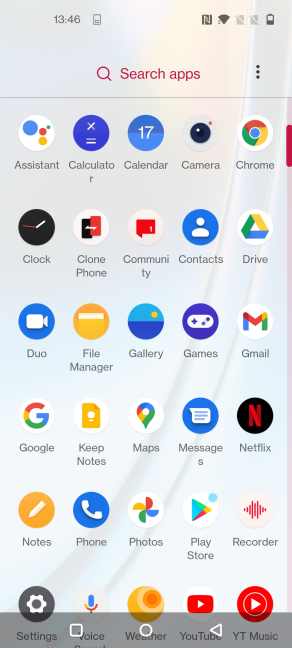The image showcases a mobile device's app search interface. At the top, highlighted in red, is the text "Search apps." Below this, a variety of app icons are displayed, providing a glimpse of the available applications on the device. Featured apps include:

- Assistant
- Calculator
- Calendar
- Camera
- Chrome
- Clock
- Clone Phone
- Gallery
- Messages
- Photos
- Phone
- Notes
- Netflix
- Duo
- Keep Notes
- Voice
- YouTube
- Games
- Community Drive
- File Manager
- Maps
- Play Store

Each app is represented by its recognizable icon, neatly arranged in a grid layout. The selection indicates a comprehensive range of tools and entertainment options, emphasizing the device’s versatility.